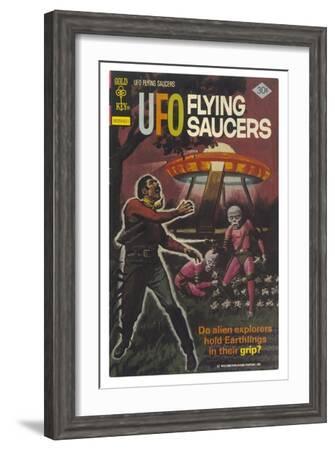This tall, rectangular framed image features what appears to be a vintage comic book or magazine cover prominently displaying a sci-fi theme centered around UFOs and alien encounters. The frame itself is composed of black wood with a white inner border, accentuating the central artwork. The top of the cover boldly reads "UFO" in three distinct colors: blue-gray, orange, and green, accompanied by "Flying Saucers" in equally large letters spread over two lines. Below this title, the scene depicts a dramatic encounter: a man with short black hair, dressed in a red long-sleeved shirt, blue jeans, and black shoes, is looking upward with arms outstretched, seemingly taken by surprise. Behind him, an orange and white UFO hovers, as though it’s either landing or already has. Two aliens are visible in the background, both donned in red uniforms, facing forward; one stands while the other appears to be on the ground. Adding to the intrigue, a tall tree with thick, dense leaves rises on the left against a sky tinted with a light burgundy hue. In the bottom right corner of the cover, a caption provocatively asks, “Do alien explorers hold earthlings in their grip?” while the top right corner indicates a price of 30 cents. The overall color palette includes vivid reds, oranges, and purples, enriching the retro sci-fi atmosphere of the scene.